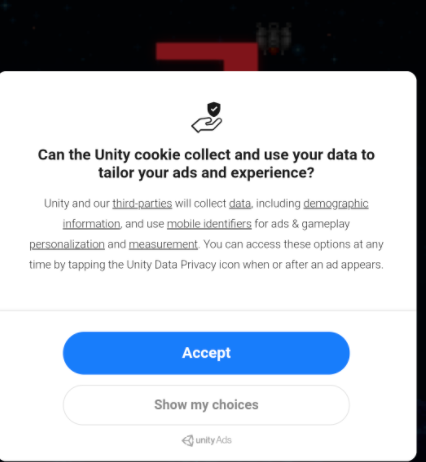The image depicts a website with a black background, featuring what appears to be a partially obscured symbol resembling the number "7" in the center. This symbol is obscured by a prominent white pop-up. The pop-up has a white background and black text, along with an illustration at the top showing a hand holding a shield with a check mark on it.

The text on the pop-up initially reads: "Can the Unity cookie collect and use your data to tailor your ads and experiences?" Following this, it details: "Unity and our third parties will collect data, including demographic information, and use mobile identifiers for ads and gameplay personalization and measurement. You can access these options at any time by tapping the Unity data privacy icon when or after an ad appears."

At the bottom of the pop-up, there are two action buttons. The first is a blue bar with white text that says "Accept." Below that, there is a white bar with black text that says "Show My Choices." Below these buttons, there is the Unity Ads logo accompanied by the text, summarizing their options to either accept data collection or view and adjust data privacy preferences.